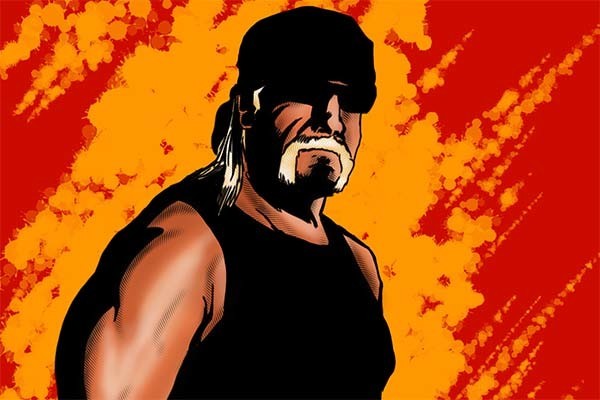This dynamic image features Hulk Hogan depicted in the stylized manner of a comic book superhero poster. The background is a vibrant gradient that transitions from fiery orange at the center, where Hogan stands, to a bold red on the edges, creating a dramatic and intense backdrop. 

Hulk Hogan is illustrated with a black beanie that is snugly pulled down to his dark shades, partially hiding his eyes. His signature blonde hair peeks out from the back of the beanie, adding a touch of familiarity to his fierce persona. His nose has a stark, heavily outlined appearance with a bright highlight along its bridge, and his distinctive blonde mustache extends downward to his chin on both sides, reinforcing his iconic look.

The fine lines etched on his face denote age and experience, while shadows under his chin enhance the depth and ruggedness of his expression. He wears a tight black muscle shirt that accentuates the impressive bulk and definition of his brawny arms and chest, emphasizing his muscular physique. Altogether, the image captures Hulk Hogan as a larger-than-life figure, exuding power and presence reminiscent of a superhero.